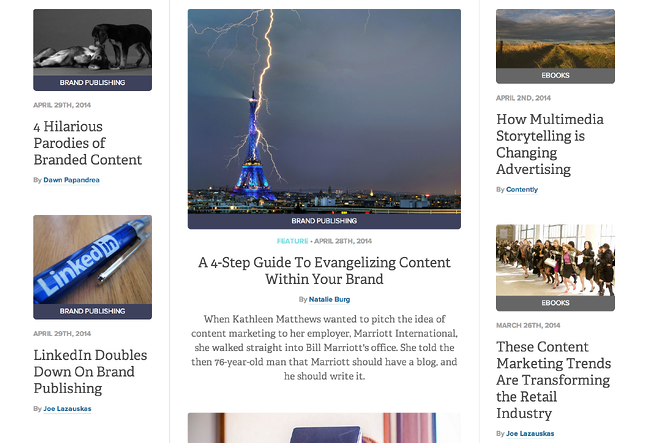On a news website showcasing various insightful and entertaining articles published on April 20th and April 28th, 2014, a series of compelling images and headlines catch the viewer's attention. 

In the upper left-hand corner, the focal point is a black-and-white photograph of a dog eating something. The headline reads, "Four Hilarious Parodies of Brand Content" by Dom Perponatsu, published on April 20th, 2014. Alongside it is a smaller image with a LinkedIn pin on a table, accompanied by a headline, "LinkedIn Doubles Down on Brand Publishing," dated April 28th, 2014.

At the center of the webpage is an electrifying image of the Eiffel Tower struck by lightning at night, illuminating the iconic structure. The article titled, "A Four-Step Guide to Evangelizing Content Within Your Brand" by Natalie Berg, dated April 28th, 2014, narrates the story of Kathleen Matthews pitching the idea of content marketing to Marriott International, convincing Bill Marriott himself of the necessity of a corporate blog.

To the upper right-hand corner, a headline reads "How Multimedia Storytelling is Changing Advertising" by Contently, displayed alongside a serene image of clouds and a vibrant orange and green pastoral landscape. Directly below this is another image showing a group of women walking in a row, illustrating a piece titled "These Content Marketing Trends are Transforming the Retail Industry" by Joe Lacoustegos.

The overall display combines striking visuals with engaging headlines to draw in the reader and offer a rich variety of informative articles centered around brand publishing and content marketing trends.